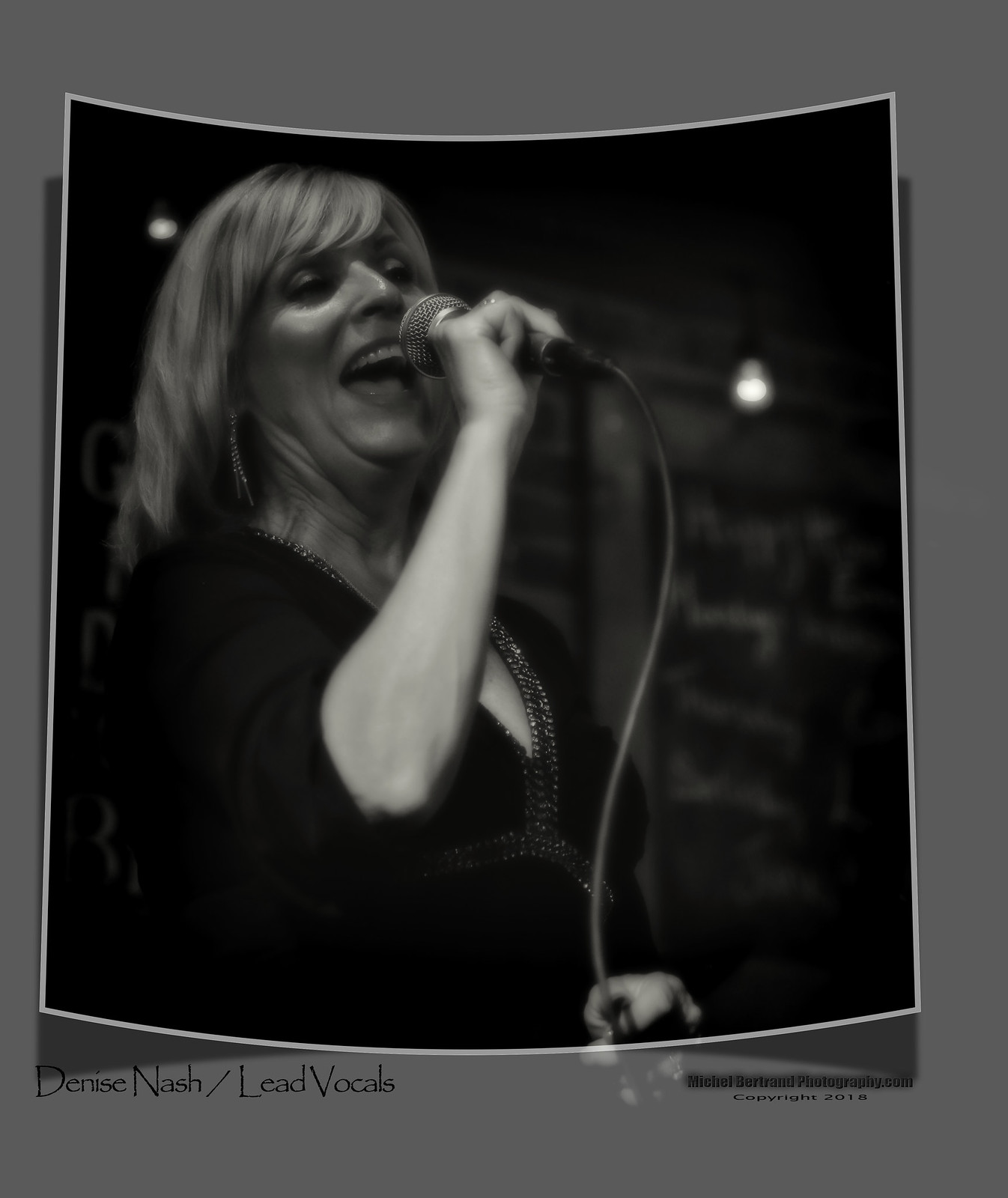This detailed black and white photograph captures Denise Nash, appearing to be in her 40s or 50s, passionately singing into a microphone. She's dressed in a black dress that features a metallic silver pattern, which elegantly extends from her neckline down to her midsection, adding an eye-catching detail. Her blonde hair cascades down, and she wears striking silver drop earrings. The photograph, evidently a printed copy curled slightly at the edges, showcases her with an open mouth and a joyful facial expression.

The indoor setting seems reminiscent of a bar, with blurred inscriptions and light bulbs visible in the blurred background, hinting at a rustic ambiance possibly characterized by stone walls and timbers. The bottom left corner of the image is inscribed with "Denise Nash / Lead Vocals," indicating her role as the vocalist, while the bottom right displays "Michael Burland Photography .com © 2018," giving credit to the photographer and the year it was captured. The printed photo rests against a gray background, adding to the vintage feel of this striking moment frozen in time.